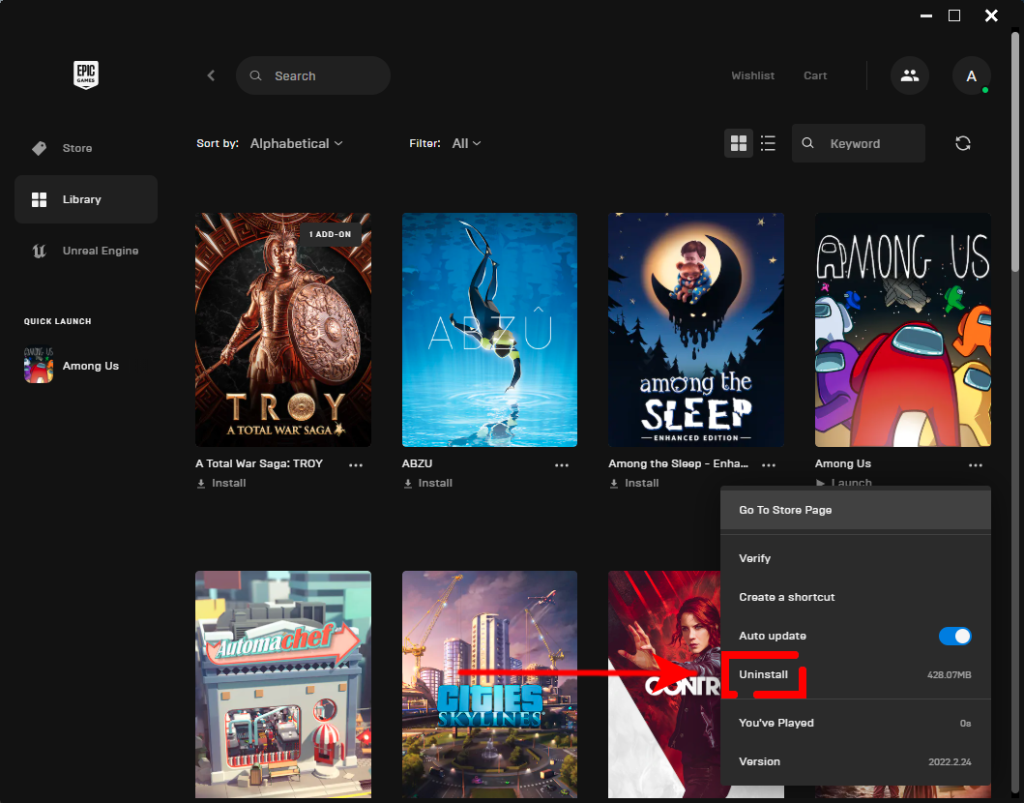This is a detailed screenshot of the Epic Games Store application interface. The background of the application is primarily black. In the top-left corner, there is a small white logo resembling a shield, containing the black text "Epic Games." Adjacent to this logo, to the right, is a medium gray search bar, shaped like an elongated pill, featuring a light gray magnifying glass on the left and the text "Search" in light gray at its center.

To the right of the search bar, separated by a generous amount of negative space, are the words "Wishlist" and "Cart" in gray text. Further to the right, separated by a thin gray horizontal line and a vertical line, is a medium gray circle icon with two white profile silhouettes. Next to this, there is a dark gray circle with a white capital letter "A" and a small red circle in the bottom right corner.

Beneath this top section is an informational row in white text. It reads "Sort By," followed by the word "Alphabetical" with a downward-pointing arrow icon next to it. After some negative space, the word "Filter" appears, followed by "All" with another downward-pointing arrow icon. Further to the right, after more negative space, there are several selection icons: a medium gray box with four white squares, and next to it, a set of three vertically-stacked white lines, each with a white dot beside them. To the right of these, there is a medium gray search box with a light gray magnifying glass inside it, containing the text "Keyword." Outside this search box, to the right, there is a white refresh icon.

Below this row, various game images are displayed. In the bottom right corner of the screenshot, a dark gray pop-up window is visible. It features the word "Install" in white text, enclosed almost entirely by a red box, with a red arrow pointing to it.